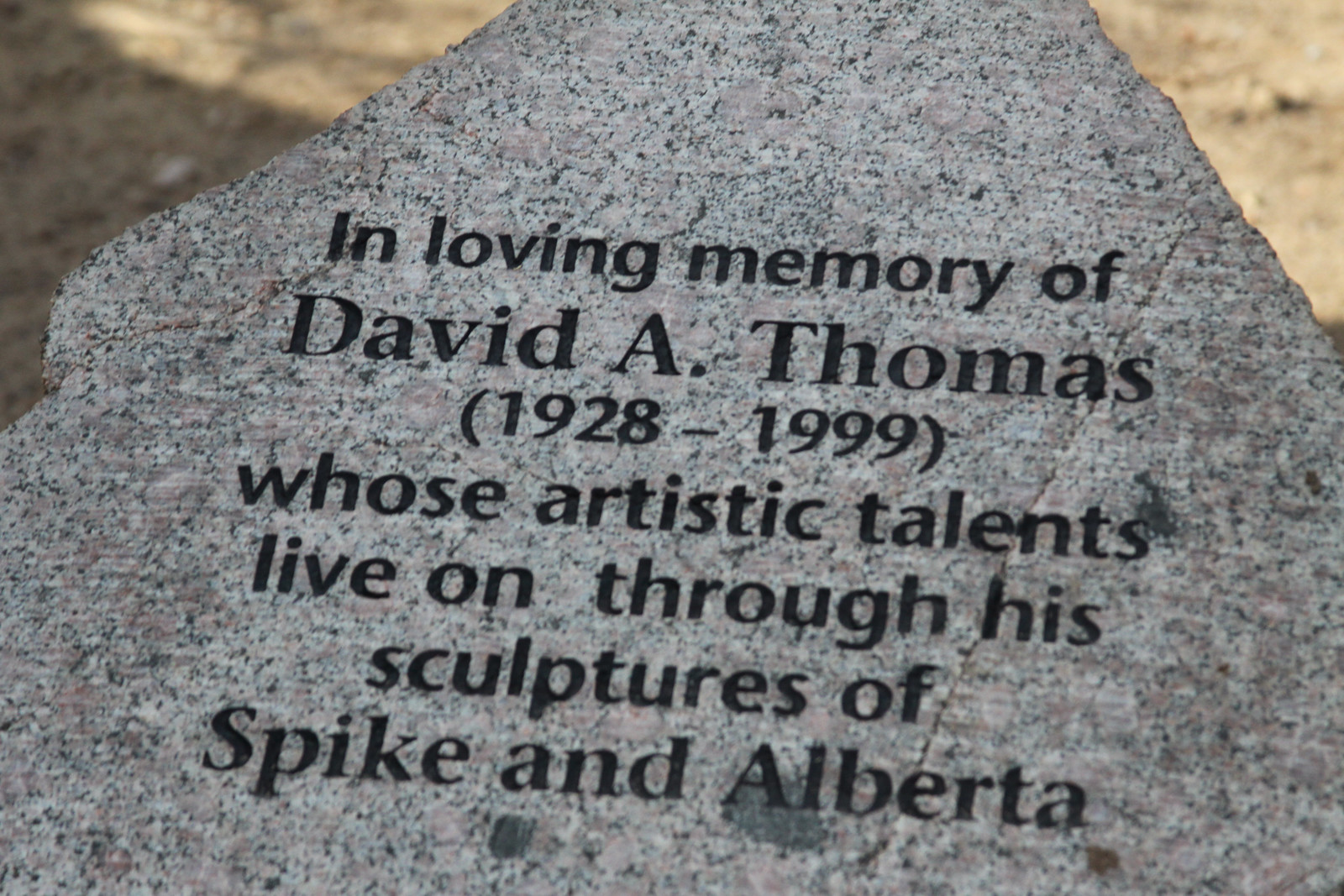This close-up photograph captures a triangular-shaped gravestone made of granite, featuring a polished gray surface dotted with dark gray and faint reddish spots. The gravestone bears a black etched inscription that reads: "In loving memory of David A. Thomas (1928-1999), whose artistic talents live on through his sculptures of Spike and Alberta." The stone stands slightly cast in shadow on the left, while the right side is illuminated by sunlight. The background at the upper corners reveals a dirt surface, devoid of the expected cemetery grass, adding a rustic element to the scene.